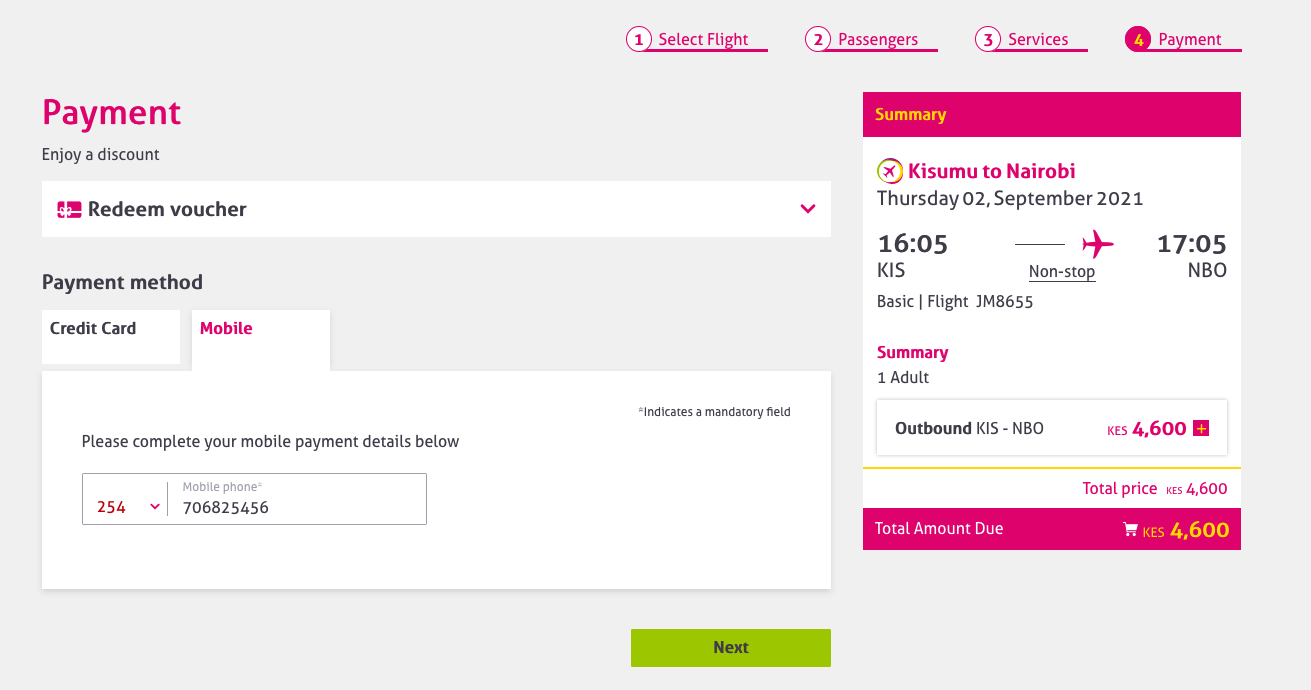**Payment Landing Page for Flight Booking**

The landing page, designed in a light gray palette, is dedicated to finalizing the payment for a flight booking. Dominating the top section of the page is a progress tracker, showcasing four steps: "Select Flight," "Passengers," "Services," and "Payment." Each step is indicated in bright pink text, with the numbers in corresponding circles. The first three steps are denoted by white circles with pink borders and numbers, while the active step, "Payment," is highlighted in solid pink with a white number 4.

Below this, a detailed summary of the payment information is displayed within a vertical white box, accentuated by a bright pink banner at both the top and bottom. The top banner reads "Summary" in gold text. Underneath, in bright pink, are the flight details: "Kisumu to Nairobi," accompanied by a flight icon. The travel dates and times are stated in black text: "Thursday, 02 September 2021, Airport KIS to NBO, nonstop, 1605 departure, 1705 arrival," with a pink airplane icon between the two airport codes.

Further breakdown of the flight details includes the flight number "JM8655" in black text, and the passenger information: "Summary: 1 Adult," also in black. This is followed by the cost summary within a light gray box, showing "Outbound KIS to NBO" and the cost of "KES 4,600." The total price is also listed as "4,600." The bottom pink banner indicates "Total Amount Due" in white text, with "4,600 KES" in gold to the right. At the very bottom, a prominent green button labeled "Next" awaits the user’s action.

On the left side, the section begins with the word "Payment" in pink at the top. Underneath, black text offers an opportunity to "enjoy a discount," alongside a white box for voucher redemption, featuring a dropdown arrow for additional options. The payment method selection follows, with "Payment Method" in black and options for "Credit Card" or "Mobile." The "Mobile" option is currently selected. Further instructions in black text prompt the user: "Please complete your mobile payment details below," directing them to enter their mobile phone number in the provided box.